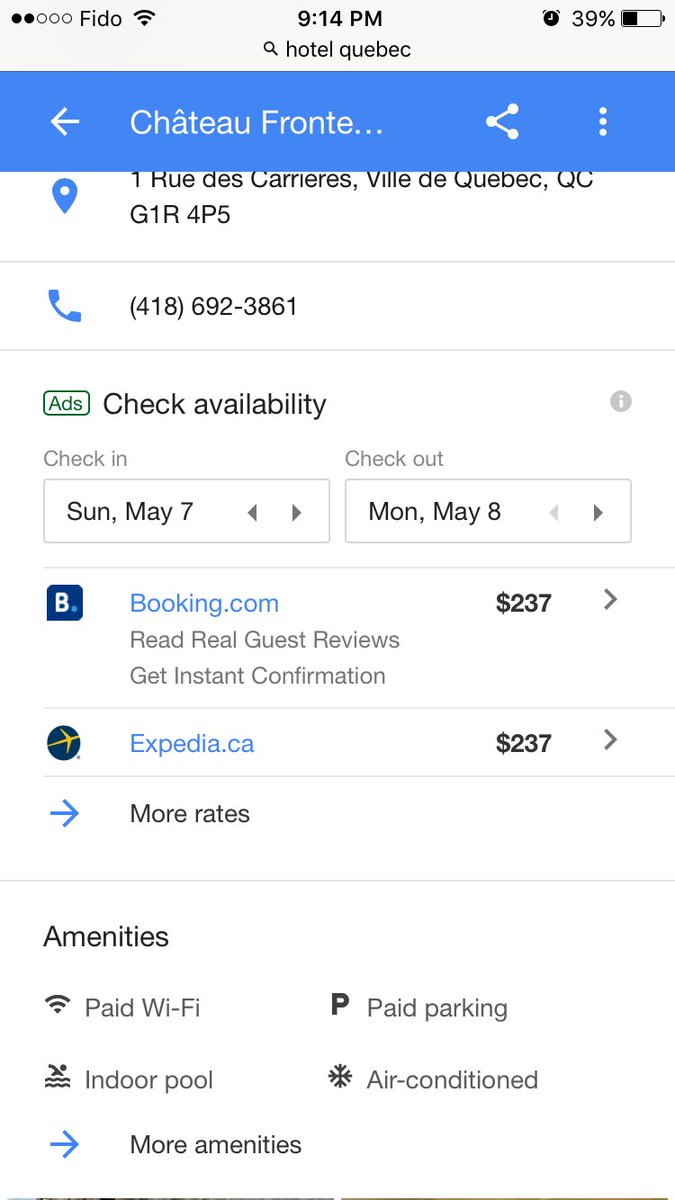The image features a web page interface that provides detailed information about a hotel search for "Hotel Quebec." At the top, a search bar confirms the query for "Hotel Quebec." Just below the search bar, set against a blue backdrop with white text, is the name "Chateau Frontier," flanked by a share button on the right, a menu button on the far right, and a back button on the left.

Proceeding downward, the main content of the page appears against a white background. It includes the hotel's address, listed as "1, Routes Carreras, Ville de Quebec, QC, G1R 4P5," and a contact phone number, "418-692-3861." 

An advertisement suggests checking availability for a stay from Sunday, May 7th, to Monday, May 8th. Below this, booking options are presented via "Booking.com" and "Expedia.ca," both offering the same price of $237. Descriptive text indicates that users can read reviews and receive instant confirmation.

Further down, the amenities are highlighted, specifically noting four features: paid Wi-Fi, paid parking, an indoor pool, and air-conditioning. Additional amenities can be viewed by selecting the option at the bottom labeled "more amenities."